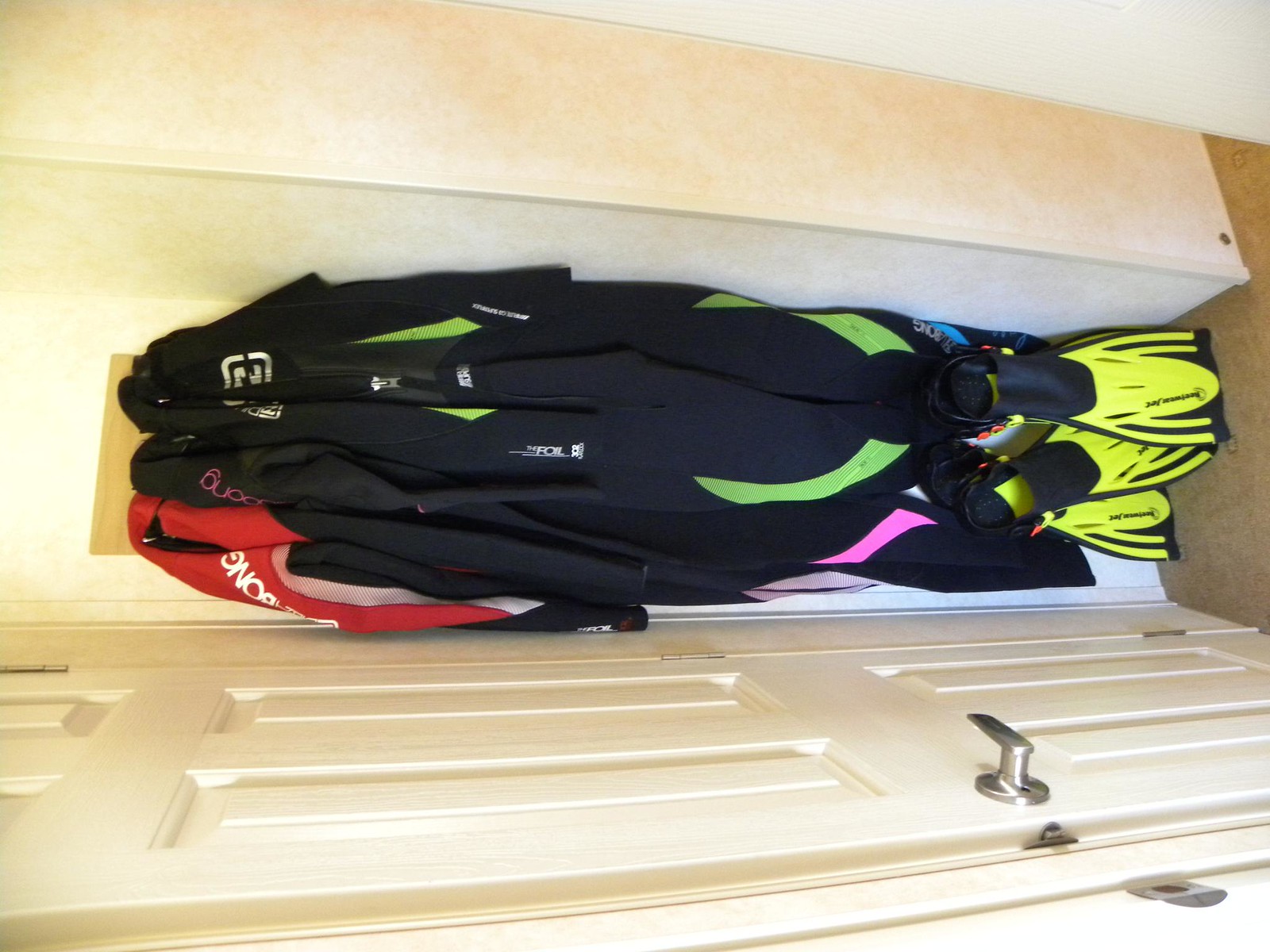The photograph is taken inside a house and shows a closet or narrow space where three black diving wetsuits are neatly hung on coat hangers. Each wetsuit features distinct colored trims: the left one has red, the middle one has pink, and the right one has green. Below the wetsuits, there are black-and-yellow diving flippers, though there appear to be only two pairs, suggesting one set might be missing. The closet has white walls and doors, with an off-white carpet. The image is rotated, giving an unusual perspective, but it clearly depicts organized scuba gear that appears ready for immediate use, situated to the left of the door, which might partially obscure them when open.